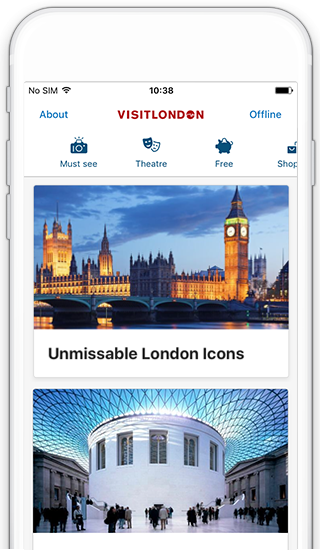The image features a white cell phone screen. In the top left corner, the status indicates "no SIM," and at the center, the Wi-Fi icon is visible. The time displayed is 10:38. On the upper right-hand side, there's an icon showing the battery status. 

At the beginning of the page, the word "ABOUT" is visible on the left-hand side in blue, capital letters. Centered on the screen, there is a large text reading "VISIT LONDON" in all capital letters and red font, with the "O" in "London" depicted as a filled-in red circle. On the left side of the screen, the word "OFFLINE" is displayed in blue.

Below this, the screen shows several menu icons:
1. A camera icon above the text "MUST SEE."
2. Two mask symbols above the text "THEATER."
3. An icon above the text "FREE."
4. The text "SHOP," which is partially cut off from the view.

Further down, there is a section labeled "UNMISSABLE LONDON ICONS," accompanied by a relevant image.